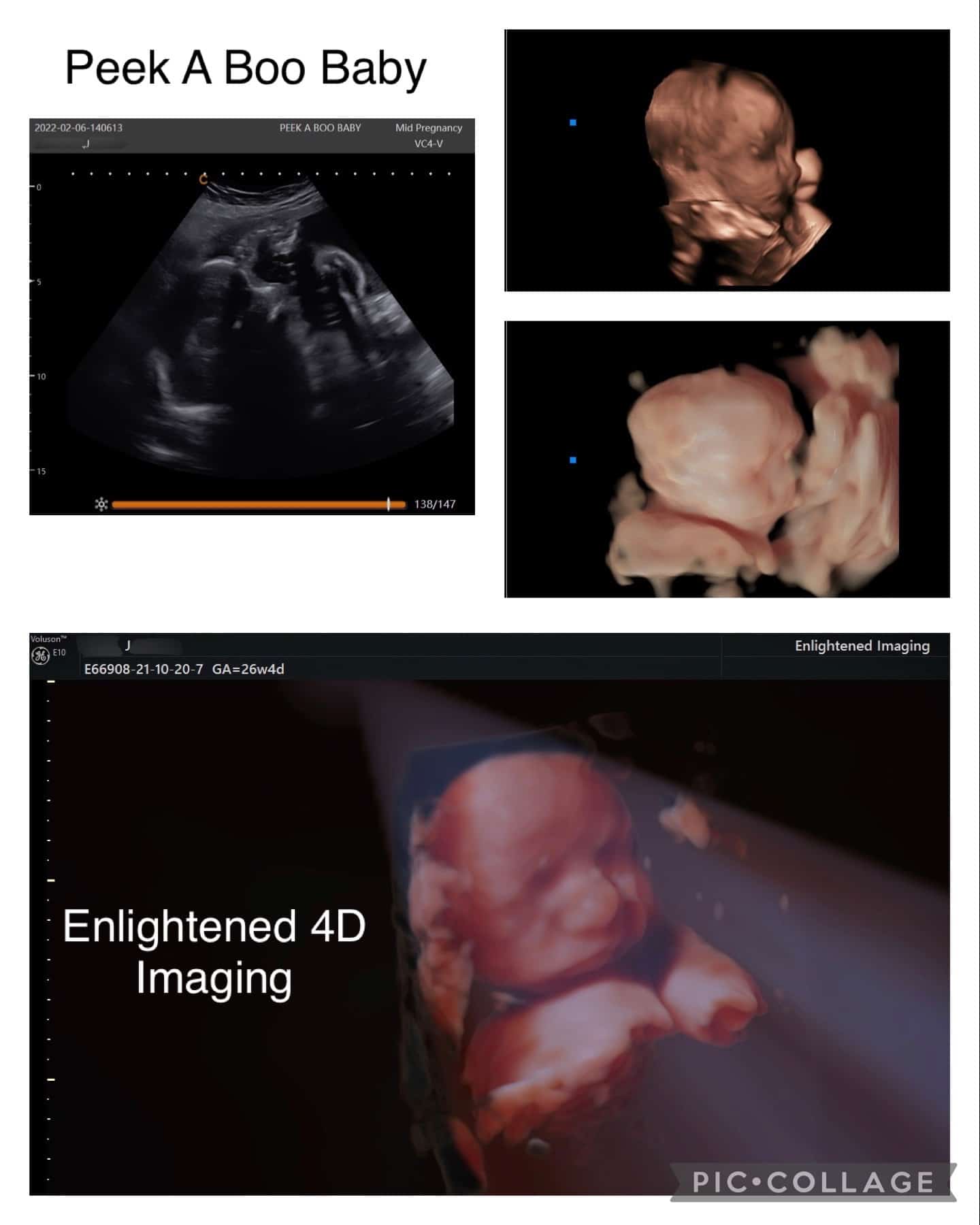The image collage consists of four ultrasound images showcasing different stages and techniques of prenatal imaging, watermarked with "PicCollage" at the bottom. In the top left corner, there's a traditional black-and-white ultrasound with the caption "Peekaboo Baby." Below it, there are two colored 3D ultrasound images stacked vertically, providing detailed views of the baby's facial features, including closed eyes and a small button nose. On the right side is a close-up 4D image in skin tones, clearly showing the baby's facial structure and hand positions, accompanied by the text "Enlightening 4D Imaging." The top left corner of the collage also includes typical ultrasound annotations with numbers and letters.